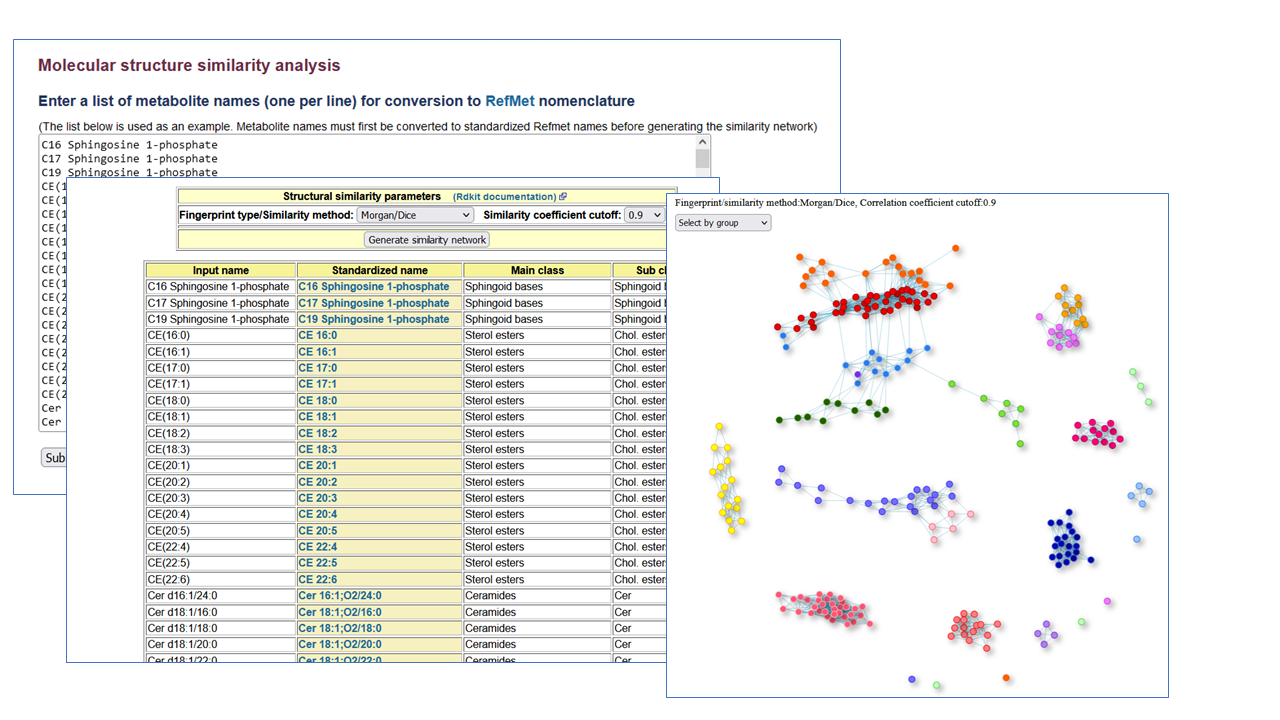The image appears to be a composite of three superimposed elements from a science or chemistry textbook, focusing on molecular structure analysis. Dominating the background are two rectangular tables or charts, one in front of the other. Each chart contains long lists of chemical names, categorized under headings such as "Input Name", "Standardized Name", "Main Class", and "Subclass". The top left table boasts a significant title, "Molecular Structure Similarity Analysis", in prominent red font. Beneath this title, smaller blue text instructs to "enter a list of metabolite names, one per line, for conversion to raffinate nomenclature," accompanied by a grid filled with numerical data, some cells highlighted in yellow and blue for emphasis.

Superimposed to the right of these tables is a square image showcasing various molecular structures. This image features colorful representations of component atoms in vivid hues of red, blue, light green, dark green, and yellow. While the molecular structures are visually detailed, the title at the top of this square image remains too small to read clearly. Each element is intricately arranged, creating a cohesive yet complex depiction of molecular data and analysis.